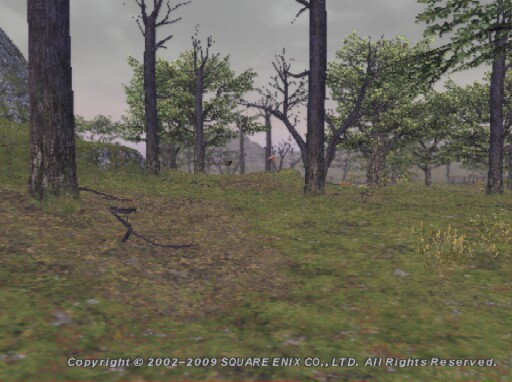Caption: 

In a serene landscape captured by Square Enix Co., Ltd. between 2002-2009, the ground is predominantly dirt interspersed with patches of green. To the right, there are delicate white and yellow flowers, while the left side is littered with scattered branches. Dominating the scene is a large, robust tree with thick, brown bark. The sky overhead is a moody gray, adding a somber tone to the photo. In the distance, a mountain looms subtly through the haze. The tree canopy at the top of the image showcases a mix of vibrant green leaves and barren branches, indicating the coexistence of both flourishing and dormant trees. The sun appears to be obscured, casting a gentle light through the network of branches. 

    
opyright notice: © 2002-2009 Square Enix Co., Ltd. All rights reserved.